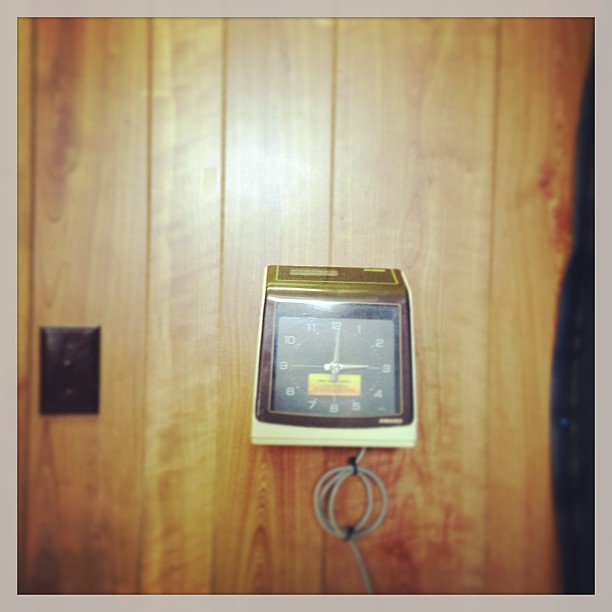This sepia-toned photograph, bordered by a medium gray frame, showcases an old wooden-paneled wall with a slightly blurred texture, likely due to age or camera focus. A gentle glare on the paneling suggests it may originate from either a camera flash or ambient lighting behind the photographer. Centrally positioned in the image is a square, boxy clock that adds a focal point with its distinct, light gray face marked by white numbers and hands. A prominent wire extends from the bottom of the clock, secured to the wall at intervals; it coils beneath the clock before straightening towards the base of the frame. A black faceplate of a light switch is also visible on the left side of the image, at the same height as the clock, adding another element of interest to this nostalgic scene.